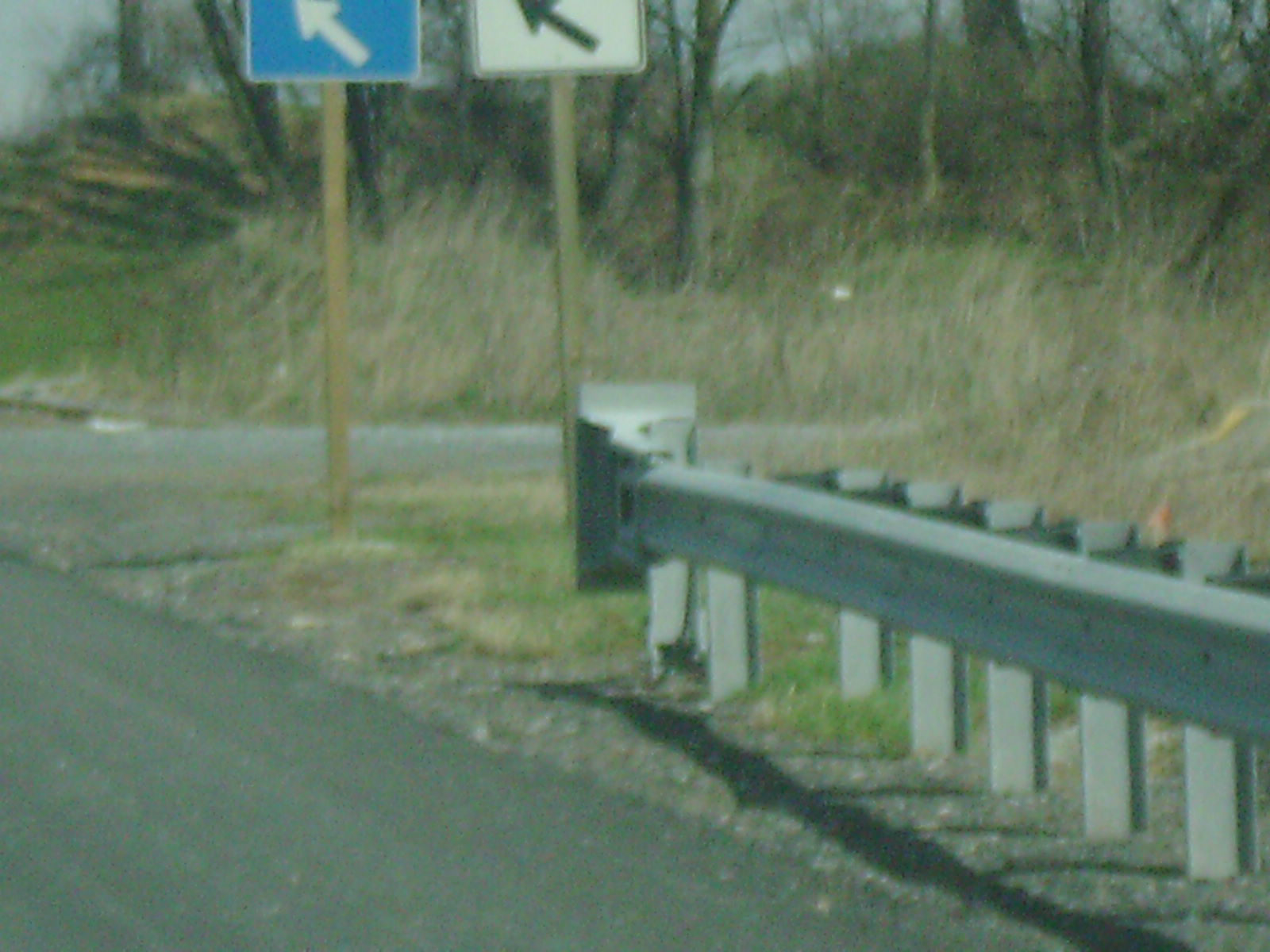This photograph captures a roadside scene prominently featuring the end section of a silver guardrail. In the bottom left corner, a gray asphalt road transitions into a gravel and rock berm. The image’s focal point is the metal guardrail, composed of silver pillars and a long strip of corrugated metal that ends around the middle of the frame. Behind the guardrail, a hillside richly covered in trees dominates the background. Midway up the hillside, patches of fresh green grass intersperse with taller, weathered grass from the previous season. Adding to the roadside details are the posts of two street signs visible just beyond the guardrail: the sign on the left is a blue rectangle with a white arrow pointing left, while the sign on the right is a white rectangle with a black arrow also directing left.